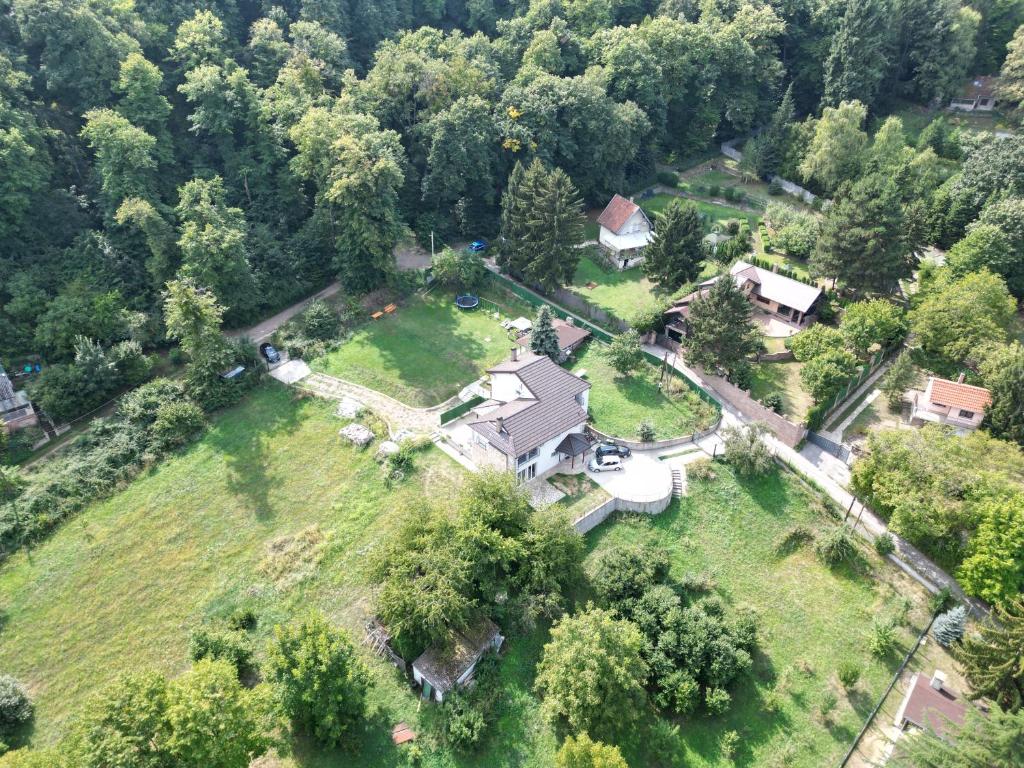This aerial photograph, taken on a sunny day, showcases a verdant landscape dominated by trees and lush green grass. At the center of the image lies a prominent two-story white house with a beige roof, significantly larger than the surrounding properties. The expansive plot occupied by this house is approximately the size of three adjacent plots combined. The driveway hosts a couple of cars, one of which is captured pulling in. To the right, three smaller, fenced-off houses can be seen, each with its well-maintained lawn and separated by roads. Dense clusters of trees and forest border the left and top edges of the image, adding to the picturesque feel. The intricate web of roads weaves through the scene, connecting the properties while no people are visible, underscoring the serene, almost idyllic, suburban setting.